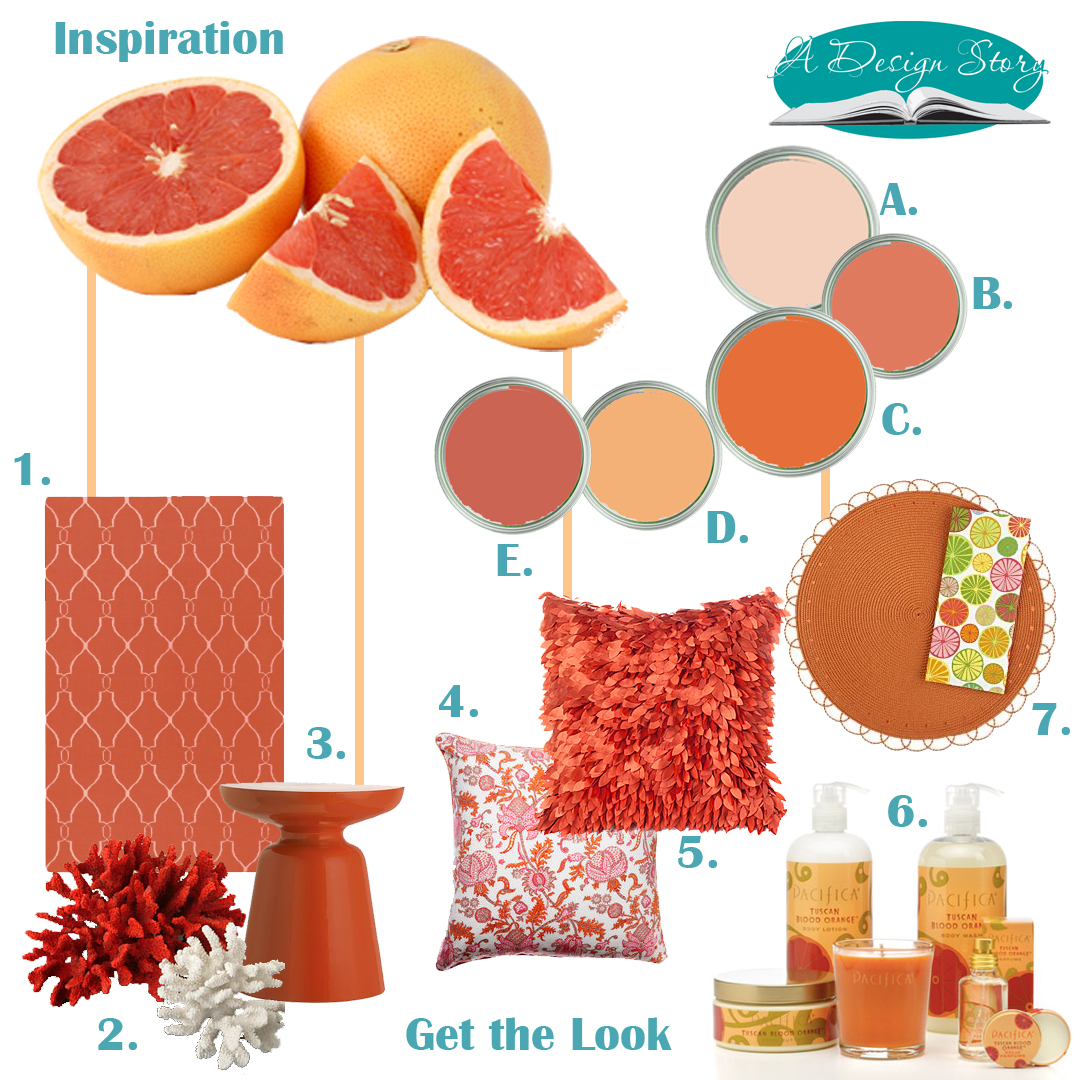The image is an infographic designed as a mood board focusing on a rustic orange-red color scheme, with various objects set against a pure white background. In the upper left corner, the word "Inspiration" is written in aquamarine, situated above a collection of oranges—one whole, one sliced in half, and two quartered. These oranges have orange lines connecting them to various similarly-colored items. In the upper right corner, within a blue oval, are the words "A Design Story" accompanied by an open book icon.

At the top, there is a grapefruit (or a similarly colored fruit) surrounded by items resembling paints or eyeshadow palettes, labeled A through E, in shades ranging from light tan, brown, orangish, dark tan, to dark red. Below this, there are two pillows—one is feathered and red, while the other is smooth with a pink and red floral paisley design.

Additionally, there appears to be a round orange placemat with a napkin adorned with wheel-shaped fruit patterns in colors like green, red, and brown. Further down, various skincare products from Pacifica with orange labels, an orange candle, some spray bottles, and a jar are organized. The mood board also features an intricate display plate potentially used for cakes or cupcakes, next to a red and white coral-like structure. The backdrop of the image includes a rusty red and white bumpy lined pattern, adding to the cohesive color theme.